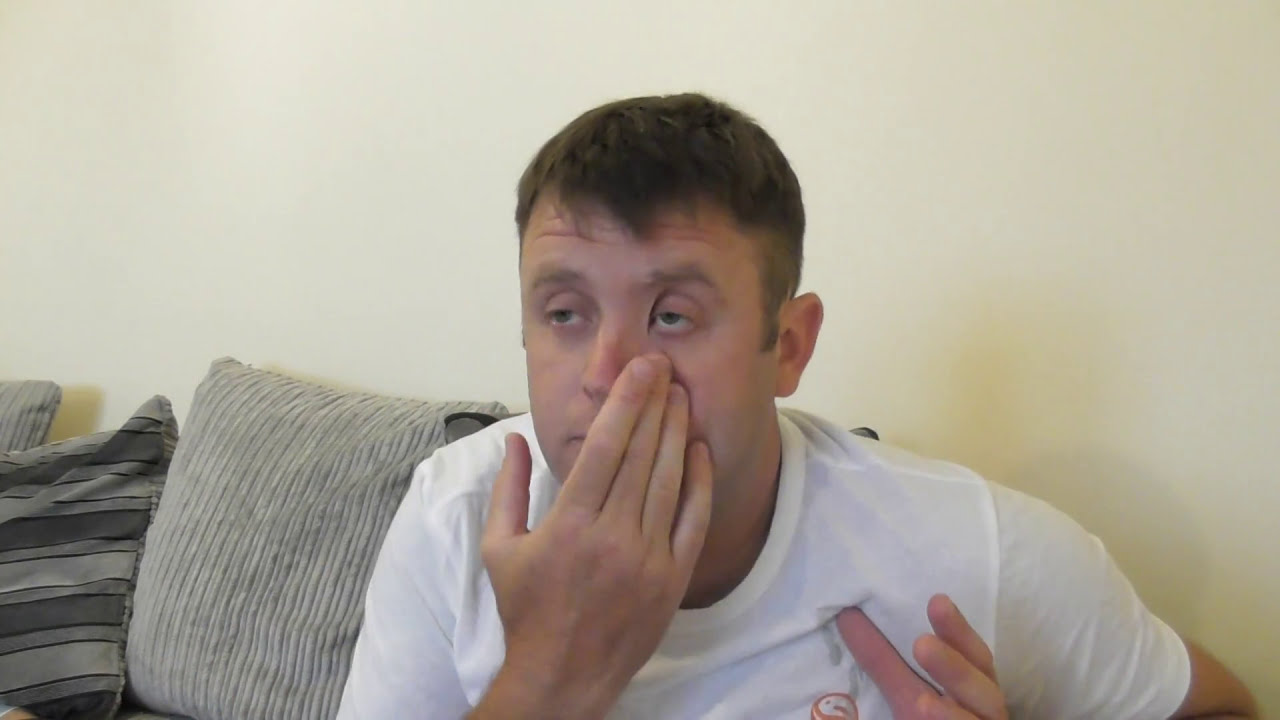A man with light skin and short brown hair styled in a military-like "high and tight" cut sits on a gray couch. The hair on the sides is kept very short while a few bangs hang over his forehead. Dressed in a white t-shirt with a small orange figure on the chest area, he holds his face with his right hand, pulling down the skin under his left eye, as if trying to remove something. His left hand rests on his shirt near the logo. The man appears deep in thought or maybe staring into space. Behind him, there are three gray throw pillows on the couch. One pillow features vertical stripes, another has horizontal stripes with various shades of gray, and the third pillow in the back is similarly gray. They sit against a cream-colored wall that has shadows cast onto it from both the man and the pillows. The overall setting provides a calm, slightly introspective atmosphere.